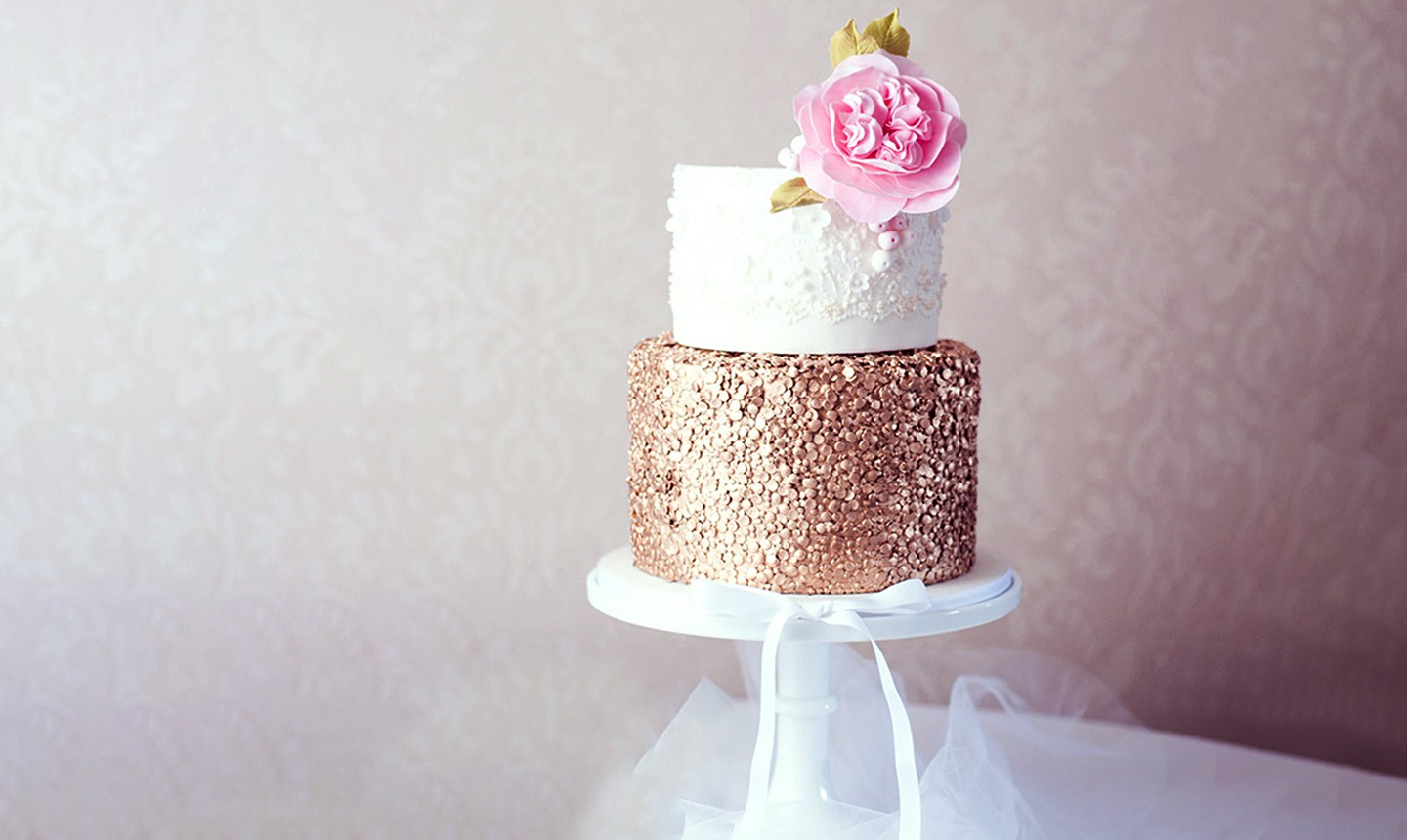This image showcases a two-tiered cake elegantly displayed on a white pedestal cake stand, which is adorned with a bow-tied white ribbon and rests atop a piece of white tulle. The background is a soft pink hue. The bottom tier of the cake is a round, chocolate cake with a grainy, crumbly texture and a shiny, golden finish. The top tier is a smaller cake iced in smooth vanilla, featuring a delicate lace design and sharing a similar grainy texture towards the top, especially on the right side. Sitting prominently atop the vanilla cake is a vibrant red rose flanked by yellow leaves, adding a touch of natural elegance to the overall presentation.